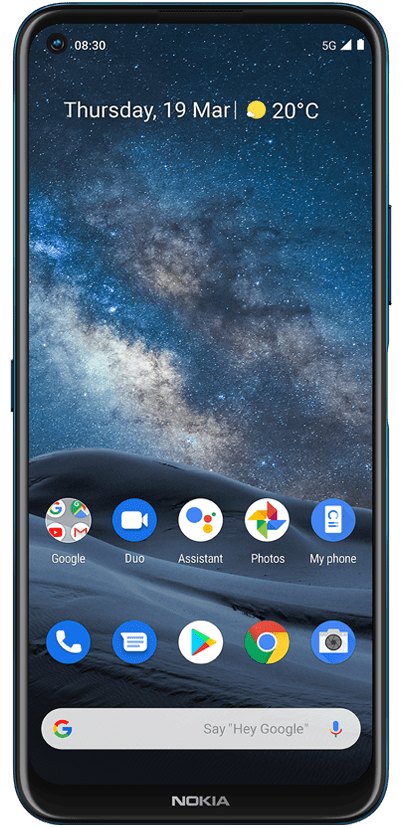Set against a pristine white background, the image showcases a sleek black Nokia cell phone. The phone features buttons on both its left and right sides. The vibrant display is adorned with an abstract, space-like wallpaper incorporating hues of black, blue, gray, and white.

In the upper left corner of the screen, the time is displayed as 8:30. The upper right corner indicates full battery, 5G connectivity, and Wi-Fi signal. Below, the screen displays the date "Thursday, 19 March," accompanied by a sun icon and a temperature reading of 20 degrees Celsius.

At the bottom of the screen are several app icons. Starting from the left, there's a Google folder encompassing YouTube, Gmail, and Google. Adjacent to it, in sequence, are the Duo app, Google Assistant, Google Photos, and My Phone. The bottom row features icons for the phone (a blue circle with a white phone), text messaging, Google Play Store, Google Chrome, and the camera app.